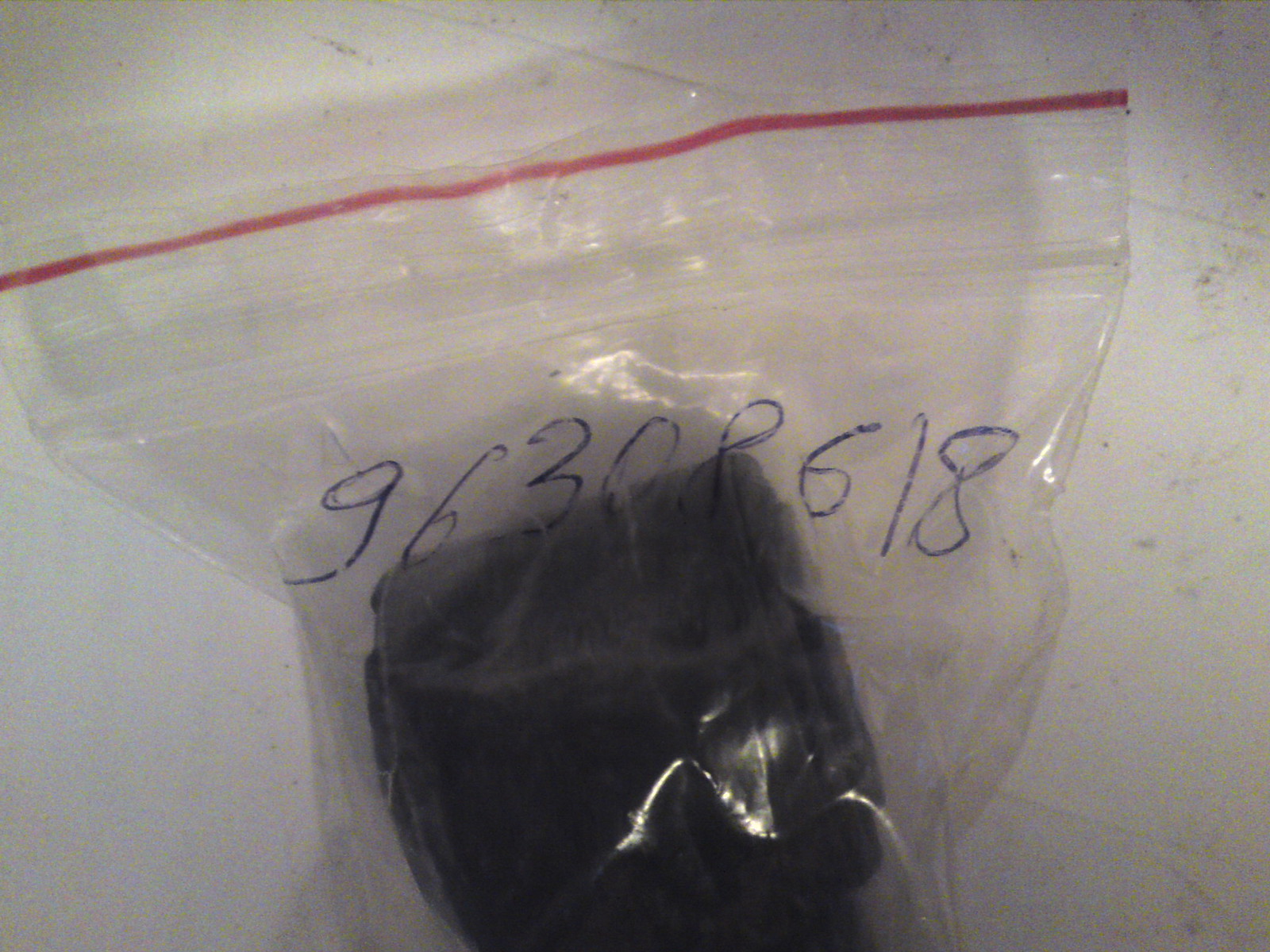The photograph, although of low quality and likely taken with an older style camera, features a small Ziploc bag lying on a flat white surface, possibly a table or a tiled floor. The Ziploc bag, characterized by its red zipper strip along the top, contains a black, cylindrical object that is difficult to precisely identify. The object could resemble a caster from a rolling chair, a lump of coal, or a rolled-up belt or wallet, suggesting ambiguity in its exact nature. The bag possesses a somewhat crinkled appearance, indicating possible reuse or prolonged storage, with numbers "96308618" written in black ink or Sharpie across its front, some of which appear slightly smudged. The overall setting seems dim or shadowy, which adds to the challenge of identifying the item inside the bag.